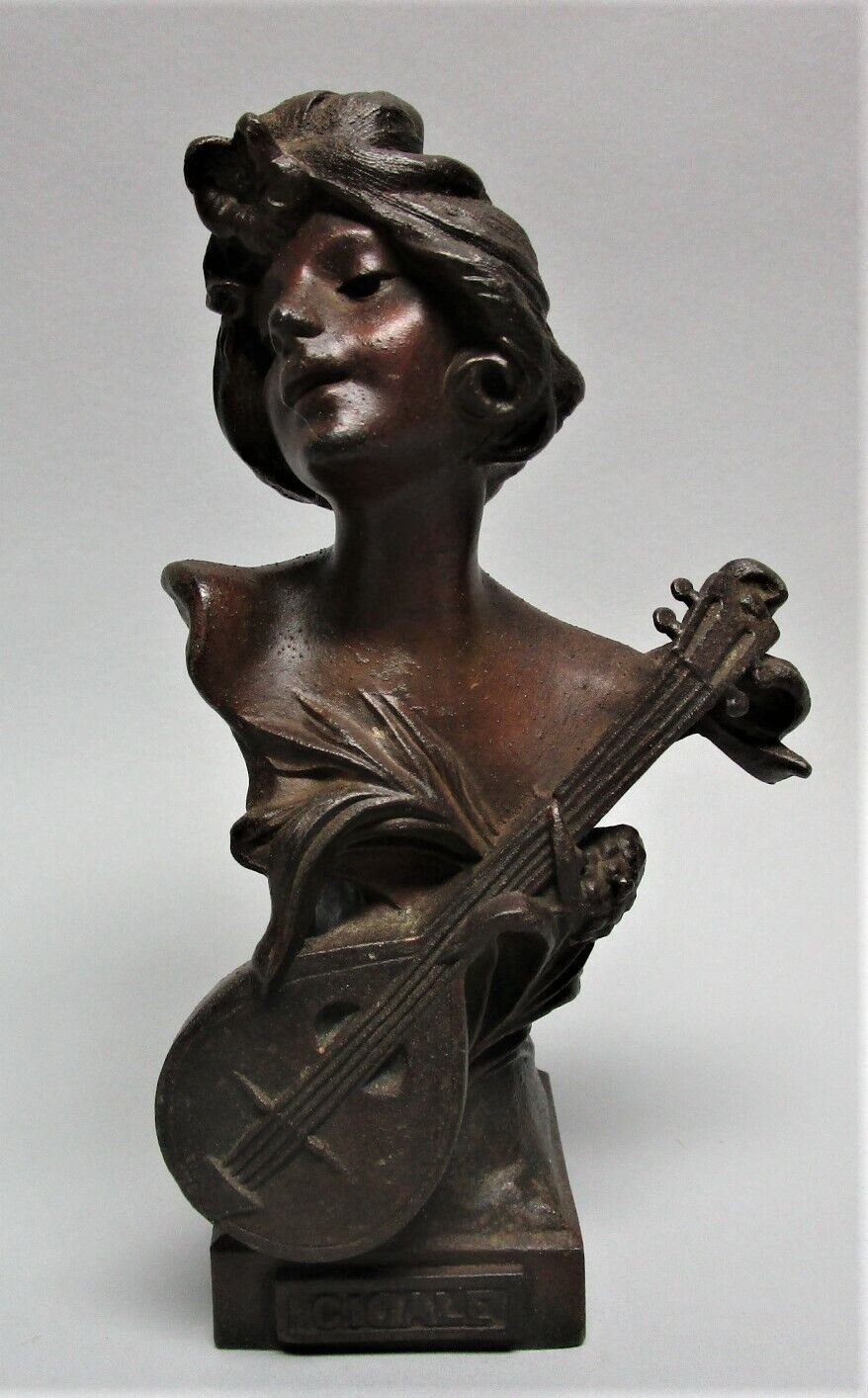This detailed image depicts a dark brown bust of a woman, likely carved from stone or molded from clay, finely showcasing an air of femininity and elegance. The woman has curly hair and is adorned with hoop earrings, with her head wrapped in what appears to be a turban or cloth that exudes sophistication. Her posture suggests she's relaxing, with her head gently tilted back. Intriguingly, despite the absence of arms, she holds a small ancient string instrument, resembling a guitar or banjo, placed tenderly against her chest. The bust is mounted on a pedestal inscribed with "CIGALE," highlighting its refined artistic presentation.